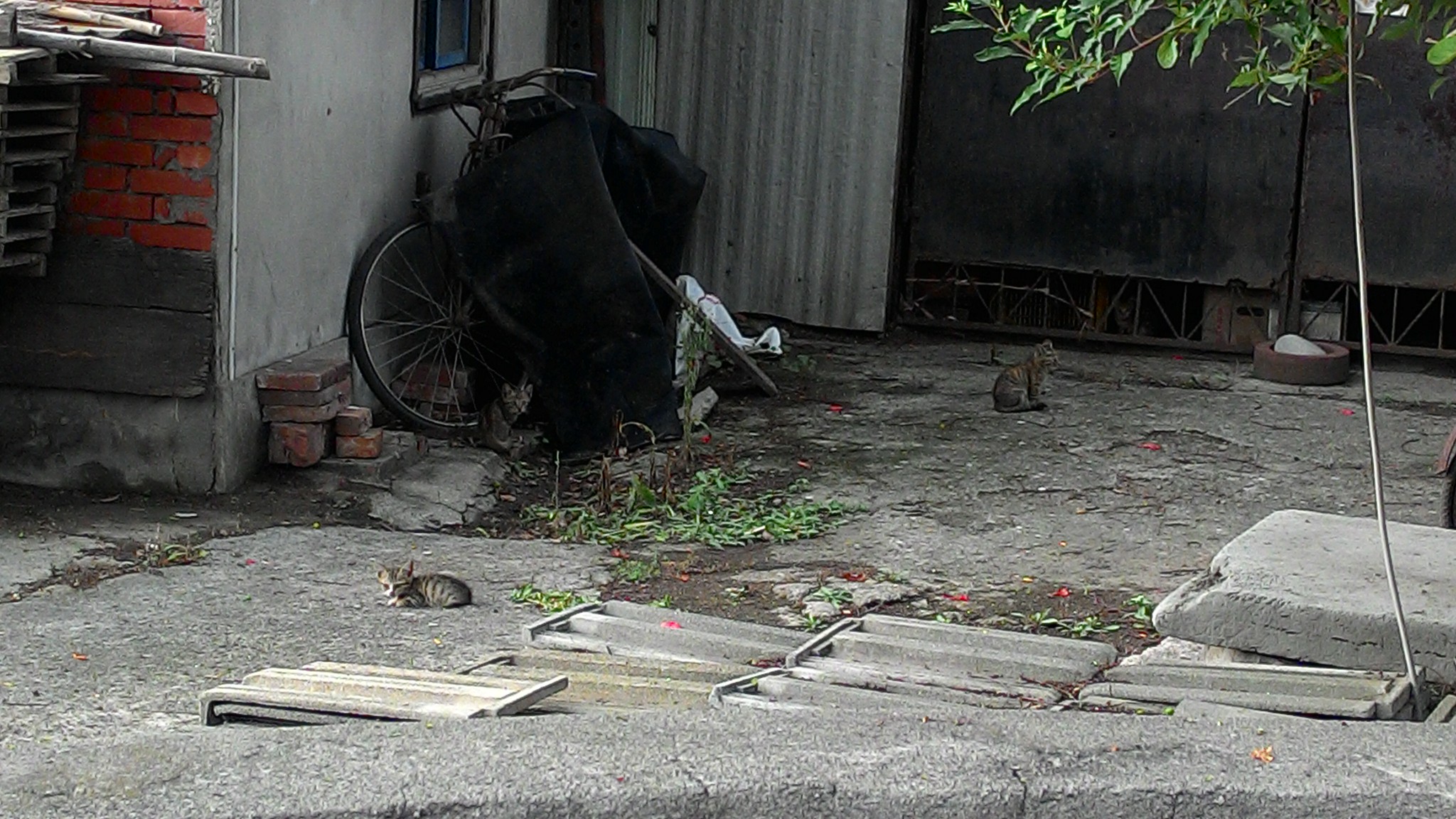The image captures a dilapidated alleyway or inlet adjacent to a sidewalk in an impoverished area, possibly within a third-world country. On the left side stands a small shack constructed from cement, rusted tin roofing, and red bricks, displaying clear signs of decay. A weathered, white wall with a small window is part of the structure, and beneath this window leans an old bicycle. The bicycle is partially covered by a black tarp or cloth, with an additional piece of white material draped over it. Scattered around the scene are several kittens: one tiny kitten lies on the cracked cement in front of the bicycle, another sits in profile looking to the right side of the frame, and a third is partially visible, peeking out from behind the bicycle. Nearby, there are sewage grates unique to the area, broken cement blocks, and stacks of bricks. The overall ground is cracked and unkept, with sparse greenery pushing through the dirt. The background reveals more of the dilapidated condition with another crumbling shack. Towards the top right, green leaves suggest a thin planted tree, adding a small bit of life to an otherwise rundown scene.